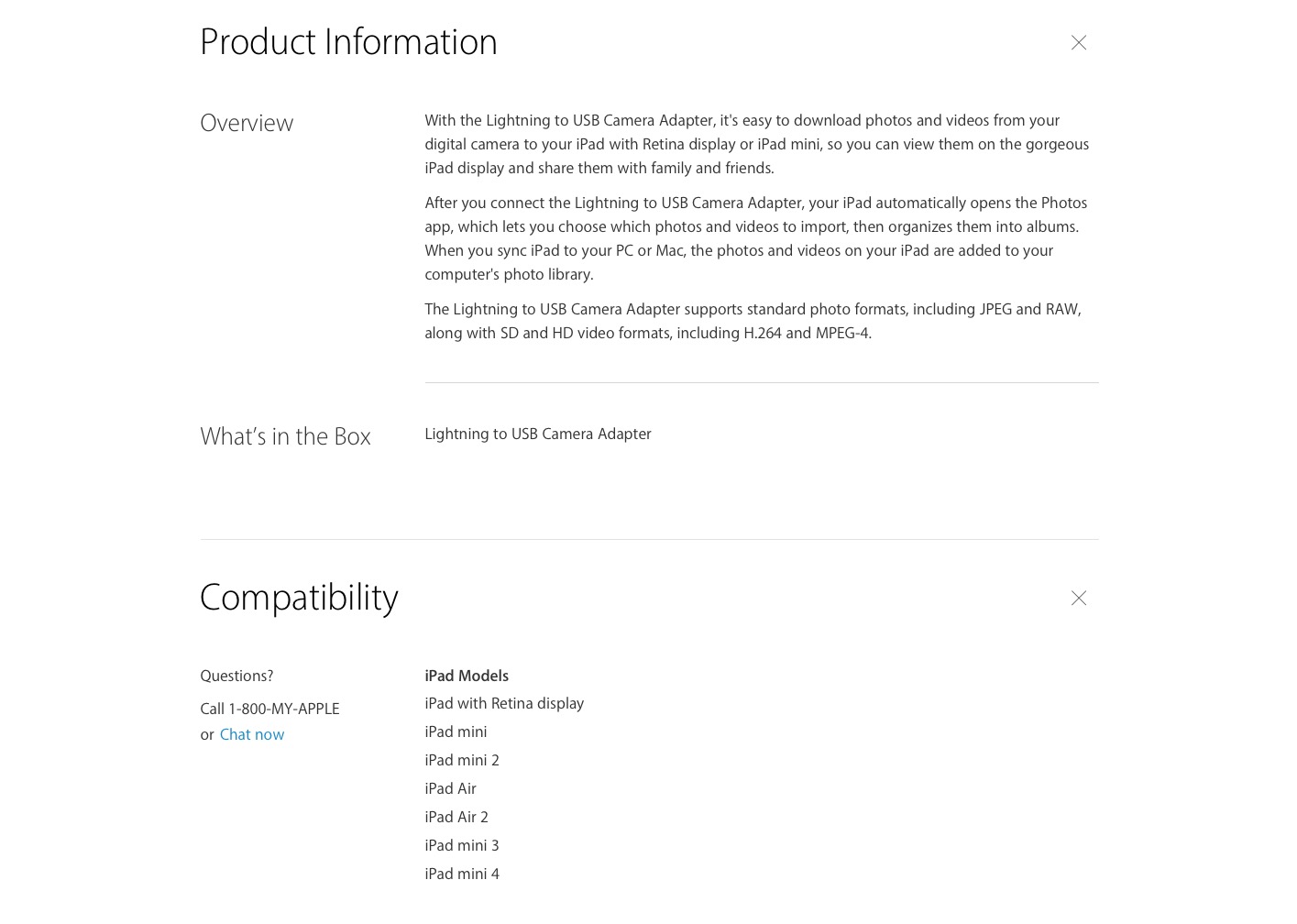Screenshot of Product Information for a USB Camera Adapter

The image is a screenshot featuring product information for a Lightning to USB camera adapter, set on a completely white background. At the top, the title text reads "Product Information." The content is organized in a two-column layout, with the left column labeled "Overview" and occupying about one-fourth of the screen. The right column, which takes up about three-fourths of the screen space, contains a detailed description split into three paragraphs.

The description states, "With the Lightning to USB camera adapter, it's easy to download photos and videos from your digital camera to your iPad with Retina Display or iPad Mini. This allows you to view them on a gorgeous iPad display and share them with family and friends. After you connect the Lightning to USB camera adapter, your iPad automatically opens the Photos app. This lets you choose which photos and videos to import and then organizes them into albums. When you sync your iPad to your Mac or PC, the photos and videos on your iPad are added to your computer's photo library. The Lightning to USB camera adapter supports standard photo formats, including JPEG and RAW, along with SD and HD video formats, including H.264 and MPEG-4."

Following this, there is a section titled "What's in the Box" which lists "Lightning to USB camera adapter." A thin gray dividing line separates this from the next panel titled "Compatibility."

Both panels under "Compatibility" are located on the left half of the screen. The top panel contains the text "Questions? Call 1-800-MY-APPLE or Click Chat Now," with "Click Chat Now" highlighted in blue text. Below this, a list outlines compatible iPad models: iPad with Retina Display, iPad Mini, iPad Mini 2, iPad Air, iPad Air 2, iPad Mini 3, and iPad Mini 4. The label "iPad models" is printed in black, and a gray "X" is positioned in the upper right corner of both the main and sub-panels for closing.